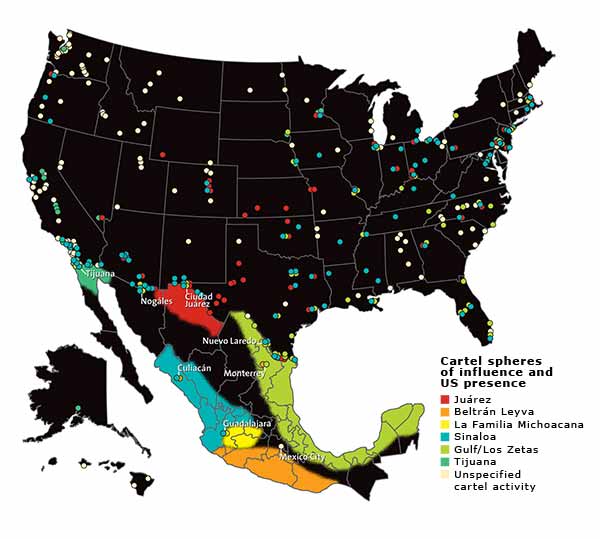This detailed image map encompasses both the United States and South America, with a specific focus on cartel spheres of influence across these regions. In the map, the entirety of the United States is depicted in black, yet the individual state boundaries are distinguishable through faint white outlines. Scattered across this black expanse are numerous dots in various colors. A corresponding key situated in the lower right corner of the map elucidates the significance of these colors: red represents Juarez cartel activity, orange for Beltran Leyva, yellow for La Familia Michoacana, blue for Sinaloa, light green for Gulf/Los Zetas, medium green for Tijuana, and white for unspecified cartel activity.

The South American map section, notable for different colored regions, provides greater detail with some marked cities. This map section also features the colored regions mentioned in the key, clearly delineating the territories dominant by various cartels. Predominantly, the cartel activities are concentrated around the eastern and western coasts of Mexico. The key at the bottom right not only categorizes these territories but also draws direct connections to the color-coded dots scattered in cities across the United States, indicating the presence and impact of these cartels within American regions.